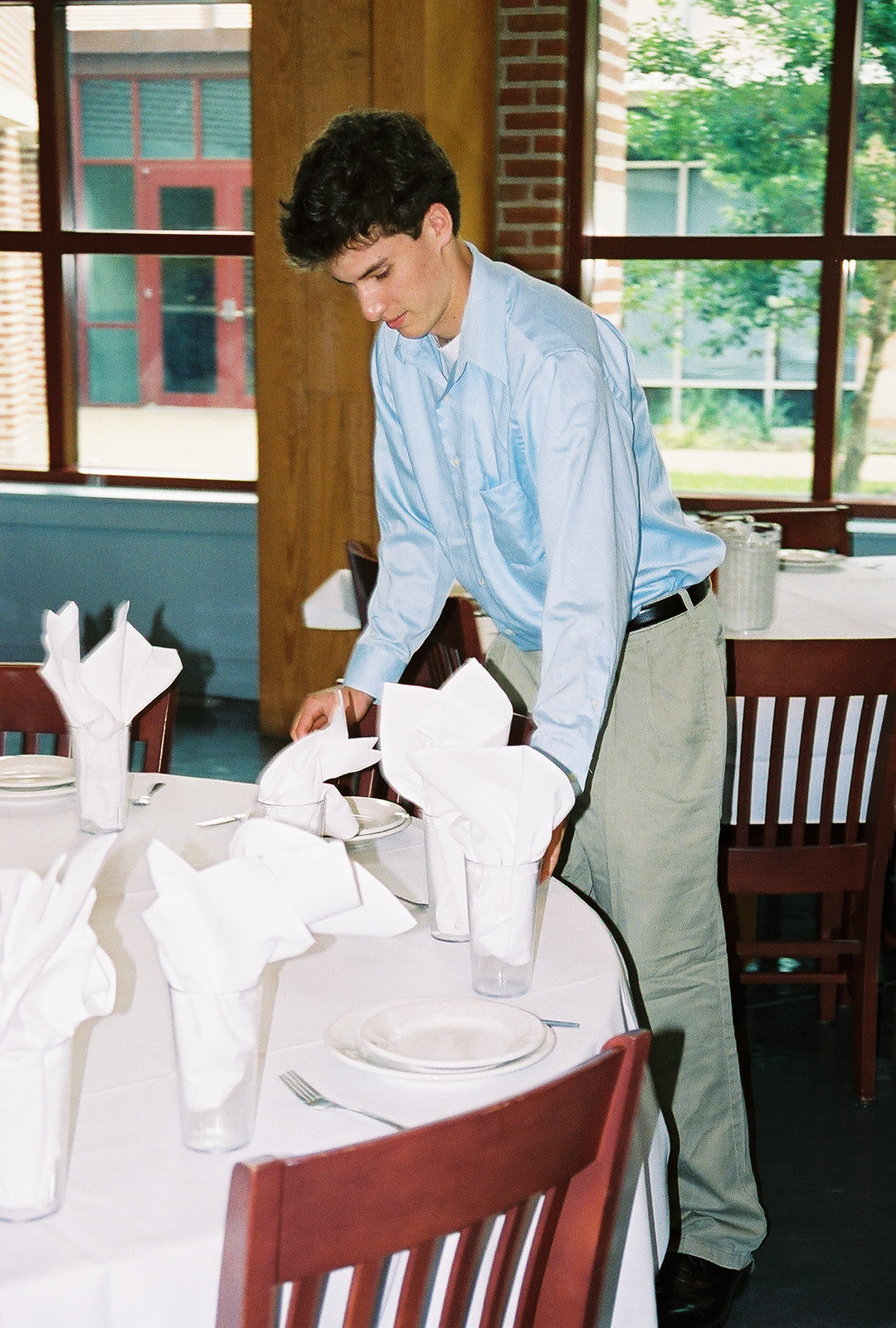This photograph captures a young man, likely in his 20s, setting up a round table in what appears to be a small, boutique restaurant or possibly a school cafeteria. He has dark brown, short hair and is dressed smartly in a light blue collared button-down long-sleeve shirt, beige khakis secured with a black belt, and black shoes. The table he is arranging features a crisp white tablecloth and is adorned with white plates, silverware (a fork on the left and a knife on the right of each plate), and clear glasses with white napkins neatly tucked inside. The young man is leaning over the table, as if placing or adjusting a napkin. Surrounding details include wooden chairs and another similarly set table in the background, with a window framed in brown through which another building is visible. There are also double doors and possibly a glimpse of a tree outside, indicating it might indeed be midday.